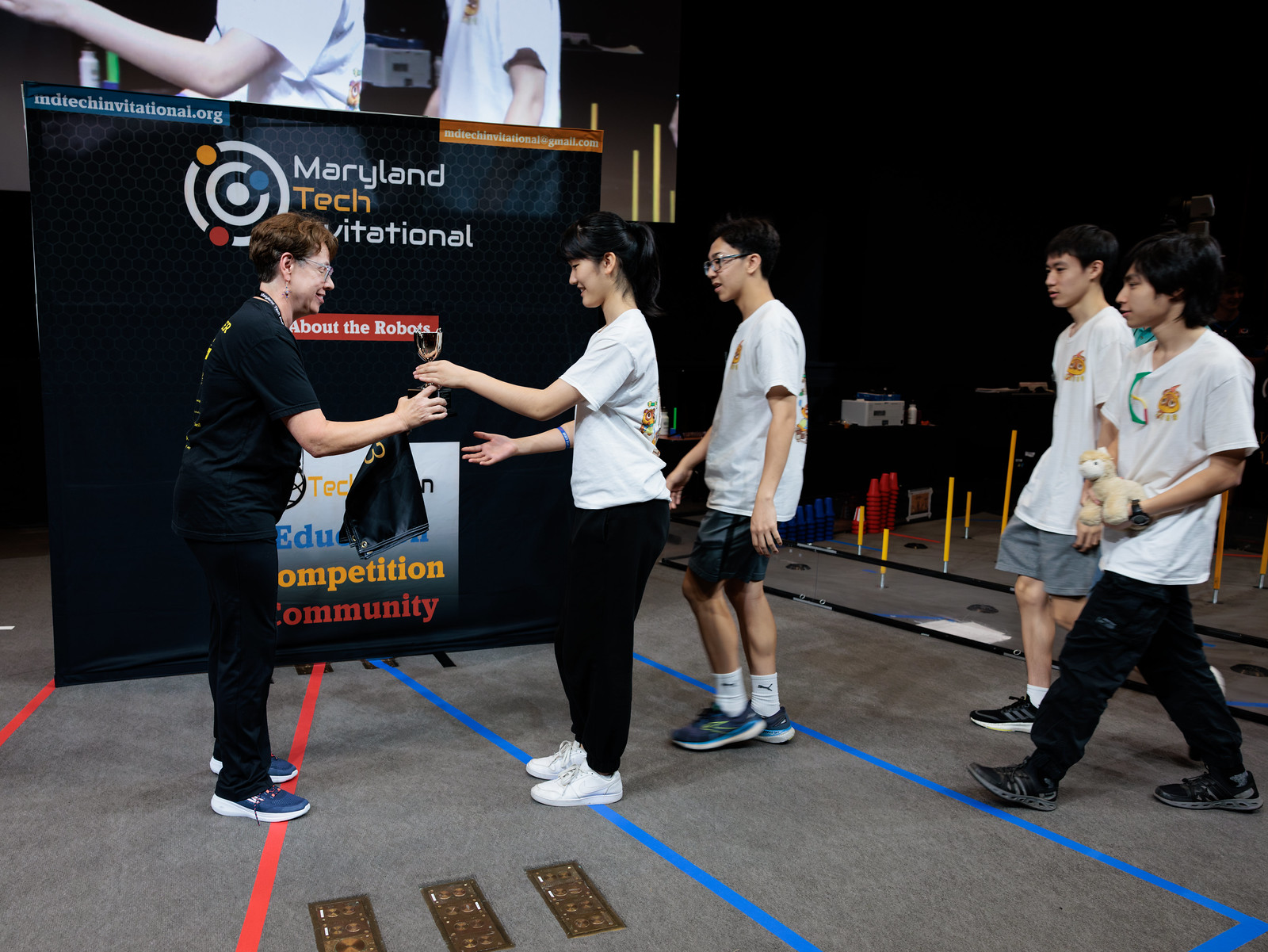In a gymnasium with a gray floor marked by red and blue stripes converging towards the back, there stands a prominently displayed poster reading "Maryland Tech Invitational" in white and gold letters, surrounded by concentric circles filled with colors like orange, blue, and red. Central to the scene is an older woman, likely in her early 50s, with short reddish-brown hair and glasses. Dressed in black sweatpants and a matching top, she reaches out with her right hand to hand over a trophy. Her blue sneakers with white rims stand out against the floor. 

Opposite her, a young Asian teenage girl in a white t-shirt, black pants, and white sneakers reaches out with her left hand to accept the trophy. Her dark hair is pulled back into a ponytail. Right behind her, slightly looking over her shoulder, is another youth with dark hair, wearing sunglasses, a white shirt, dark shorts, and blue sneakers. Following them are two more young Asian men; one holds a stuffed animal and is dressed in dark pants and a white shirt, while the other wears gray pants and a white shirt. 

The scene appears to depict an award ceremony at an educational event, likely linked to robotics, given the visible words and context on the poster behind the group. The spacious gym atmosphere hints at an organized, yet intimate event, dedicated to recognizing the achievements of these participating youths.